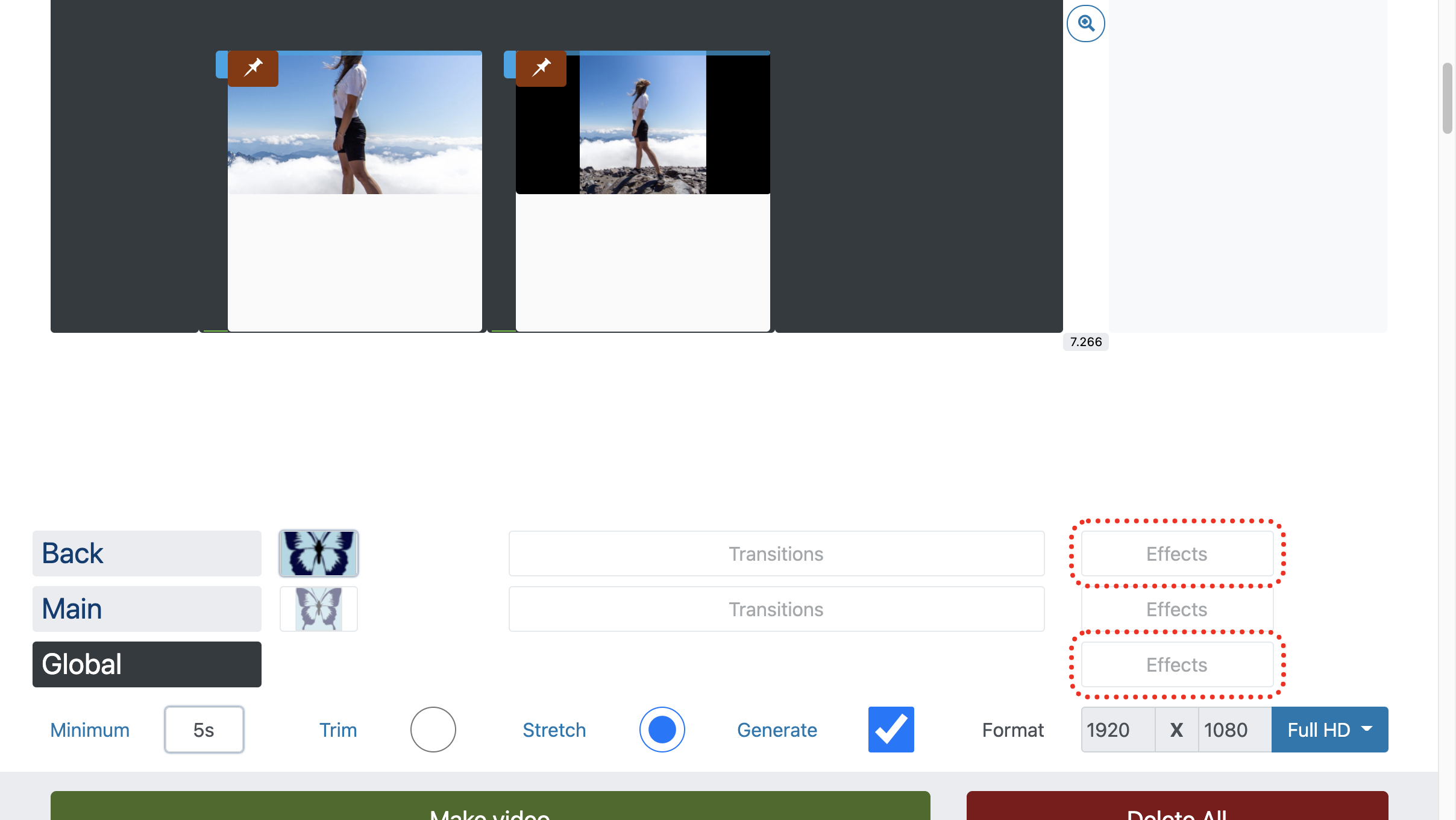The image depicts a photo editing website interface. At the very top of the interface, within a gray rectangular header, there are two square images of the same woman—a white lady dressed in a white blouse and black shorts. The backdrop in the images initially appears to be clouds, but it’s actually a beach scene, with sand beneath her feet and water stretching out behind her.

The first image is a closer shot, focusing more on her upper body, whereas the second image is a full-body shot showing her entire figure against the beach background. Both images are bordered in black.

Below these two images, the interface offers multiple tool options and settings for editing photos. There are buttons for navigating back, labeled "Main" and "Global," and various controls for image manipulation, such as to minimize, trim, or stretch the picture using circular icons.

Users can select actions with a checkmark to generate effects or modifications. One specific feature is labeled "Rex," highlighted with a red outline. Another section offers format options, including adjusting the picture's dimensions; the example provided shows a dimension of 1920 by 1080 pixels, marked with a blue rectangle labeled "Full HD."

Additionally, there are green-outlined buttons labeled "Make Video" and "Delete All," which provide functionalities for video creation and mass deletion. Overall, the interface is equipped with various tools to edit and customize photos for users.